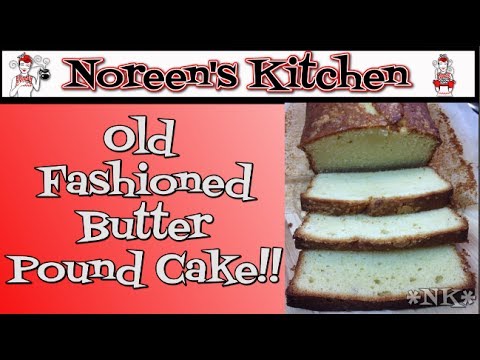The image is a detailed video thumbnail featuring a loaf of old-fashioned butter pound cake with three splayed slices, showcasing the soft ivory-colored inside and brown crust of the cake. The background features a red-to-pink gradient that transitions from left to right with white funky text, outlined in black, reading "Old-Fashioned Butter Pound Cake." Centered at the top, a white rectangular banner with a black outline and an Asian woman's figurine at each end bears the title "Noreen's Kitchen" in black serif font with a white outline and red outer glow. Additionally, two asterisks surround the letters "N" and "K" in the bottom right corner, near one of the bread slices. The overall layout is horizontal, framed by black bars at the top and bottom, giving it a clean, focused appearance evocative of an advertisement or flyer.